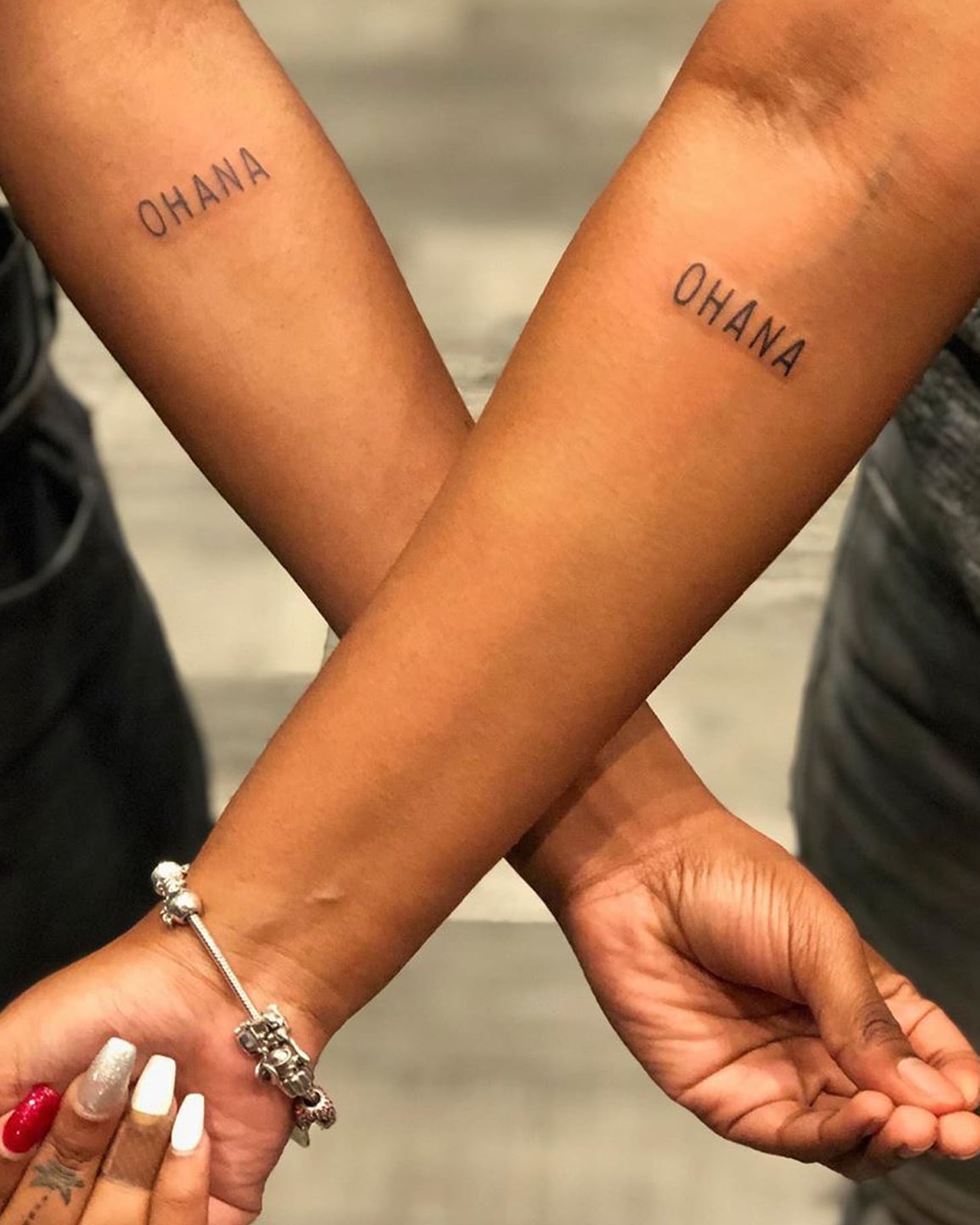This detailed photograph features the crossed forearms of two individuals, highlighting their matching "OHANA" tattoos displayed prominently below their elbows. Both tattoos, rendered in simple line art, appear fresh, indicated by slight swelling around the letters. The individuals have tan skin—suggesting they are people of color—and are wearing black and gray pants against a light gray background. The woman’s left arm stands out with its acrylic nails painted in a distinct color scheme: red on her index finger, silver on her middle finger, and white on her ring and pinky fingers. She also sports a silver bracelet adorned with various trinkets. In contrast, the other person's right arm is more understated, with natural nails and no accessories. The shared tattoo symbolizes a connection between the two, despite their contrasting styles.